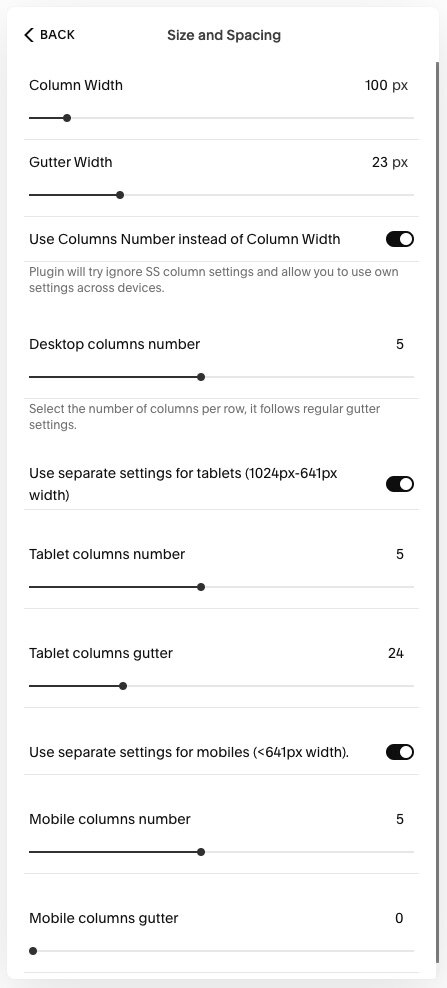This screenshot captures the "Size and Spacing" section of a settings menu from a designer layout tool. The background is predominantly white, giving it a clean and straightforward look.

In the top left corner, there's a "Back" button in bold black letters. Centered above the menu content, the heading "Size and Spacing" is prominently displayed. 

Below this heading, on the left side, the text "Column Width" appears with "100 PX" on the right side, next to a plus symbol. A slider bar beneath this text extends horizontally across the screen but is slightly adjusted towards the right.

Following that, the label "Gutter Width" appears with "23 PX" to its right, accompanied by another slider bar, similarly adjusted towards the right side.

Next, the option "Use column numbers instead of column width" is visible and selected. Under this, the text "Desktop columns number" shows a setting of "5". The next option, "Use separate settings for tablets," is turned on. 

Under this, "Tablet columns number" is set to "5", followed by "Tablet columns gutter" which is set to "24". 

Further down, the option "Use separate settings for mobiles" is enabled, displaying "Mobile columns number" set to "5". However, the last option, "Mobile columns gutter," is cropped out of the screenshot.